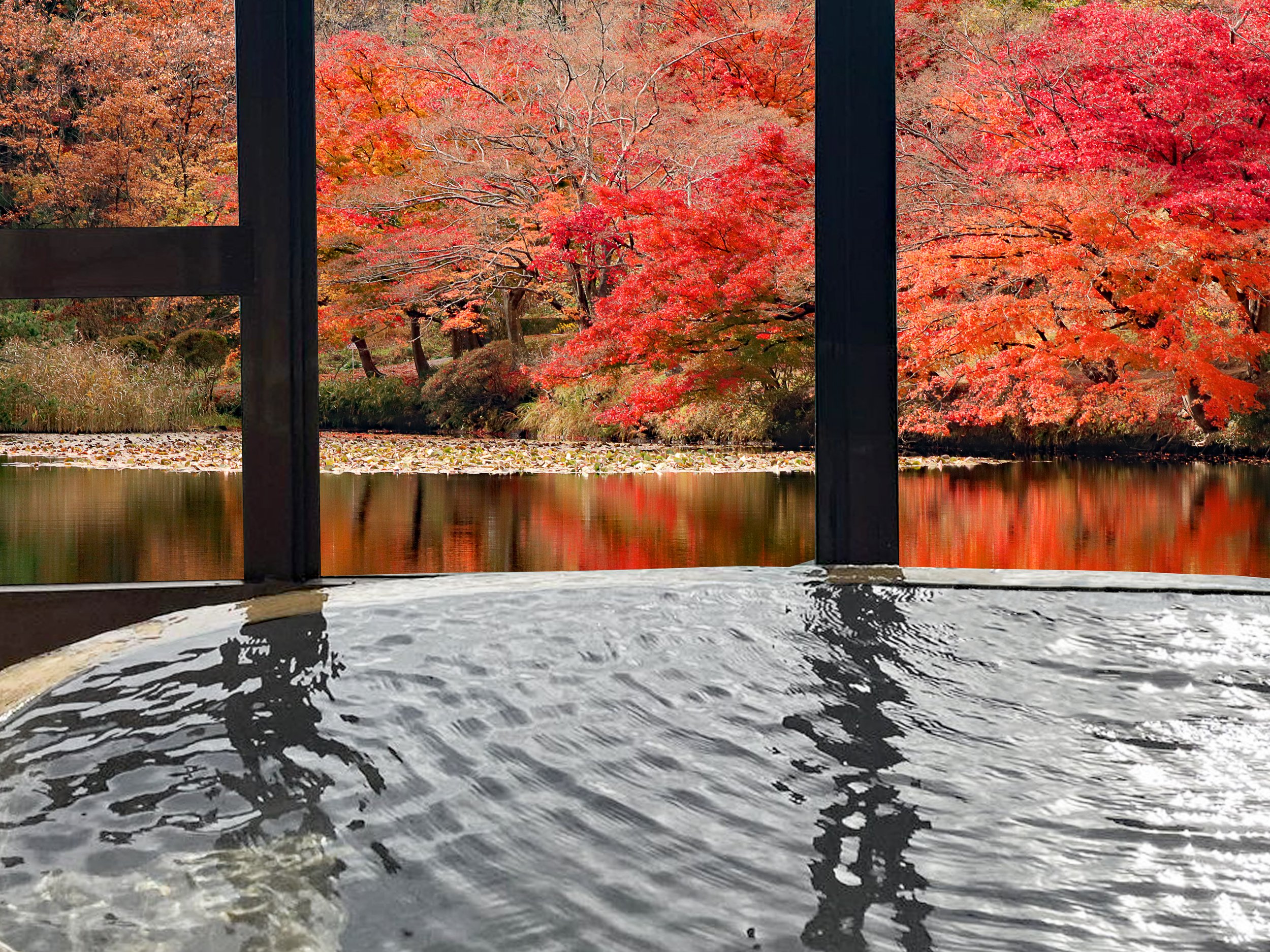The photograph captures an indoor setting with a fountain in the foreground, where the water appears murky gray and is contained within a structure supported by brown wooden posts. The scene looks outwards towards a serene lake, which is partially covered with fallen red and yellow leaves. Beyond the lake, a dense wooded area with multicolored trees—predominantly red, orange, and yellow—stretches into the distance. The image has a layered composition with multiple wooden structures: vertical pillars on the sides and a horizontal beam intersecting them. The water in the fountain appears to be standing, almost like it's overflowing, lending a tranquil yet slightly chaotic feel. The overall style is naturalistic, capturing the contrasting elements of a man-made indoor space and the vibrant autumnal landscape outside.